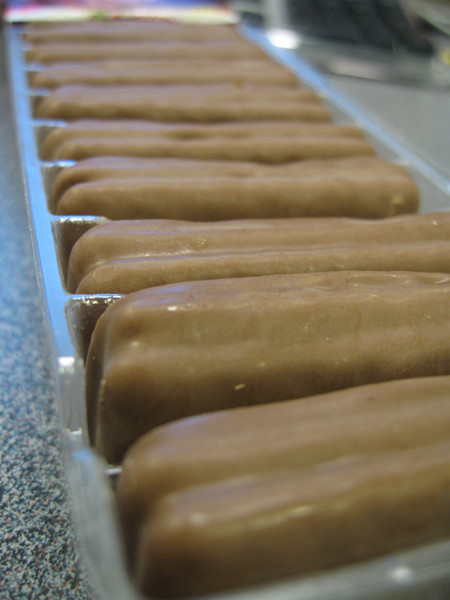This is a drab color photograph showcasing a close-up view of what appears to be a significant number of maple bars, commonly referred to as long johns or cream sticks. The pastries are arranged neatly in a clear plastic tray, typically used for packaging cookies or pastries, suggesting they are ready for sale or distribution. The maple bars are long, thin, brown, and glazed, resembling hot dogs in buns, albeit more appetizing and donut-like in appearance. The tray is placed on what seems to be a gray, tweed-like carpet, contributing to the overall industrial feel of the setup. The image is slightly out of focus, and there are some indistinct elements in the top right corner. The metallic gleam of the tray implies an assembly line setting, reinforcing the impression of mass production. Despite their somewhat plain presentation, the maple bars appear coated in a delicious layer of maple frosting.